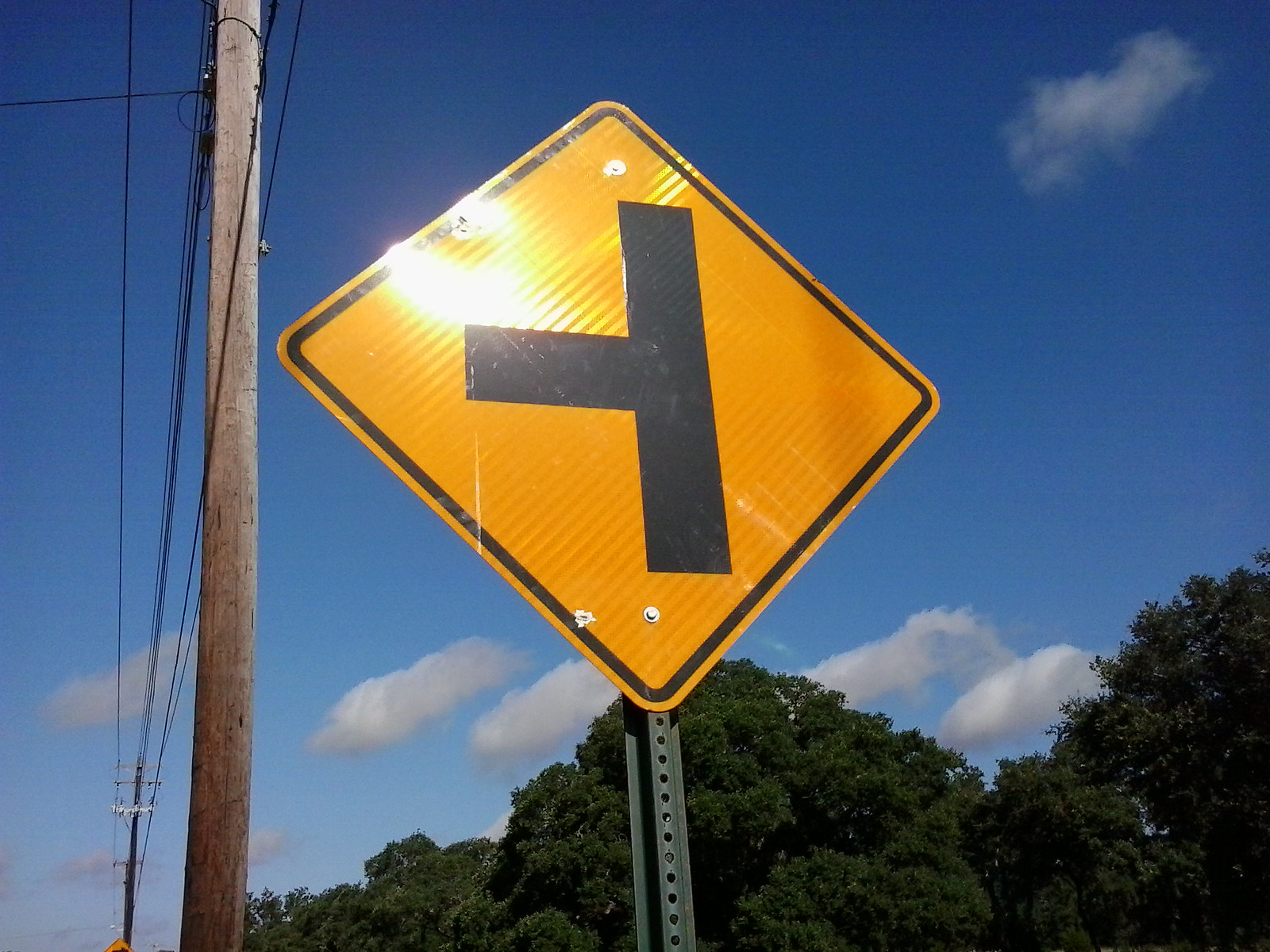This photograph captures a bright yellow diamond-shaped street sign with a black border, prominently displaying a black sideways 'T' symbol, representing a straight road with a left turn. The sign is mounted on a green metal post, characterized by circular holes along its length. This scene is set against a vivid blue sky dotted with wispy white clouds, with the sun casting a bright light in the upper left corner of the image. In the background, lush green tree canopies can be seen, providing a vibrant natural backdrop. To the left of the sign, a tall brown wooden utility pole with black electrical lines runs vertically through the entire image. Additionally, in the lower corner, there is a glimpse of another yellow road sign.